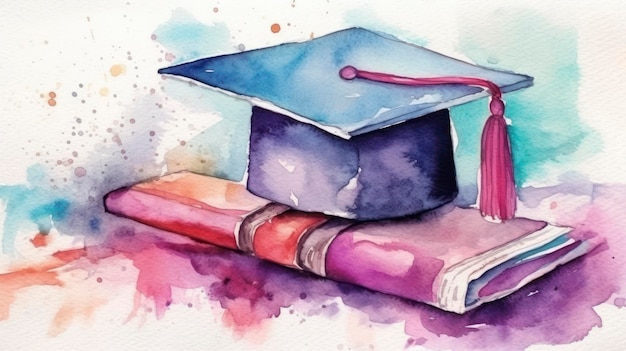The image is a detailed watercolor painting, presented in a landscape orientation and narrow-wide format. The main focus is a dark blue graduation cap with a pink tassel, positioned prominently at the top center of the painting, with the corner of the board facing the viewer. Beneath the cap lies a folded document, adorned in warm hues of pink, red, orange, and purple. The document, potentially representing a diploma, contrasts beautifully against a surface featuring a light purple wash with watercolor effects, concentrated on the bottom left and splashing along the left section. The background is a vibrant mix of aqua, light blue, pink, orange, and purple shades, adding depth and interest to the composition. This artistic piece captures the essence of graduation through its vivid and dynamic use of color.